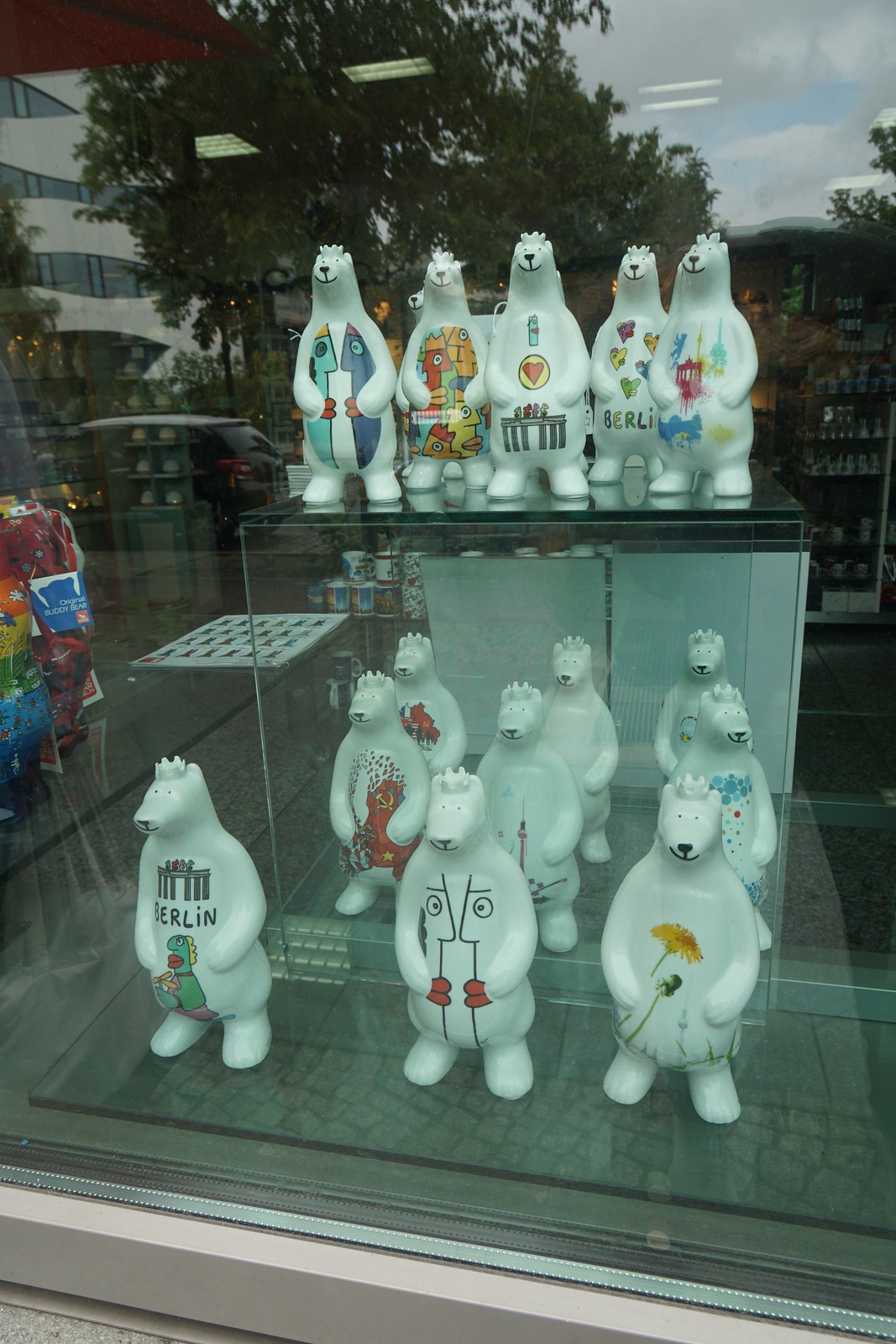In this image, we see an array of charming, cartoonish ceramic polar bear statues displayed in a store window. Each bear is crowned with a little white crown and features a unique, colorful painting on its belly, with smiles on their faces. There are six bears positioned on top of a glass display case, six inside the case, and three in front of it. Notably, the bear on the left has "Berlin" written across its stomach, hinting at the city's influence on their designs. In the background, through the window, you can discern reflections of trees and a building against the sky, further reinforcing the scene's Berlin setting. Additional details inside the shop include various shelves holding items such as t-shirts, teapots, and mugs, contributing to the vibrant and inviting atmosphere of this storefront.